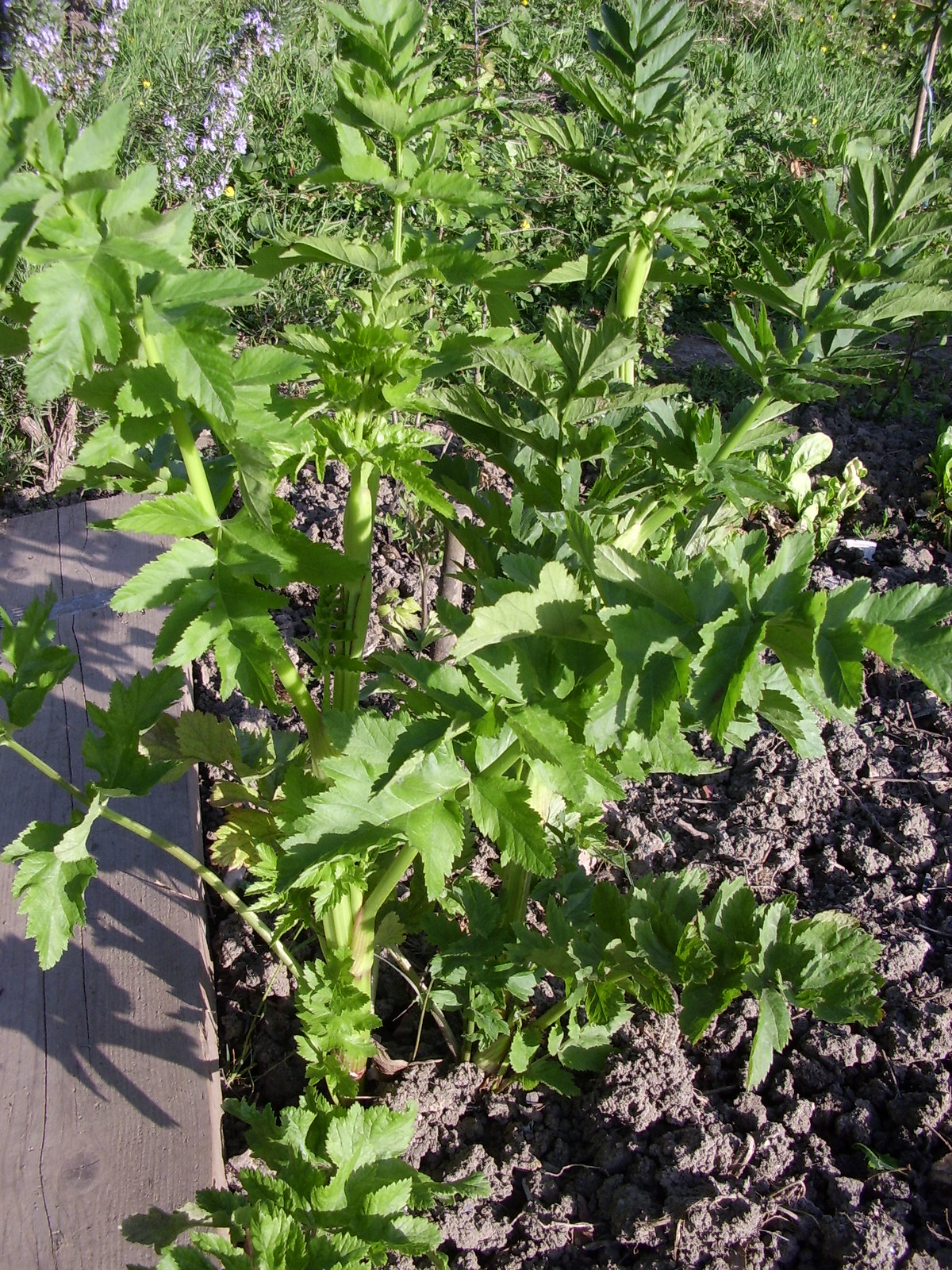This image showcases a lovely scene of green leafy plants, standing tall with round, sturdy stems that branch out robustly. The leaves are pointed with slightly jagged edges, contributing to the lush greenery. The soil beneath these plants is visibly churned and brown, indicating it's not flat or hard but rather rich and loose. Various other plants are visible in the background, some adorned with lavender-colored flowers. A light brown piece of wood with noticeable cracks runs along the left side at the base of these plants, suggesting it may have once been used as a makeshift path through the area. The overall scene, likely captured on a sunny day, features early spring growth amidst a mix of new and old leaves scattered on the ground, hinting at a possibly tranquil yet mosquito-prone setting next to an old deck or structure.